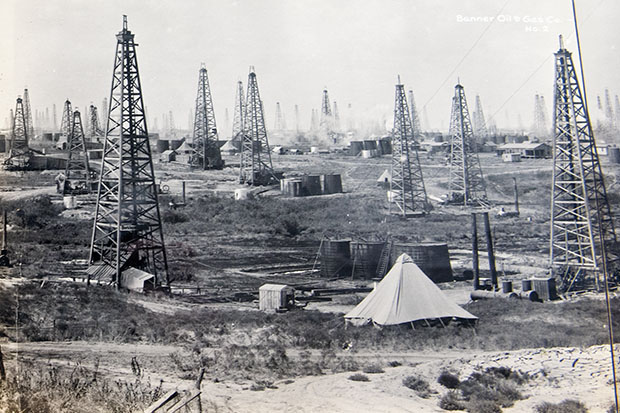This black-and-white photograph, likely taken in the early 20th century, depicts an expansive outdoor scene of an oil field. The landscape is densely populated with dozens upon dozens of metallic oil towers, resembling electrical towers in shape, which extend from the foreground into the distance, gradually diminishing in size. A light gray sky forms the backdrop, adding to the historical ambiance of the image. The ground area is a mix of sand, dirt, and small gray-hued plants scattered throughout. Prominently situated near the bottom center-right is a white tent, surrounded by various other structures including shacks, sheds, and large barrels presumably for storing oil. Dirt pathways meander between the towers and these structures, creating a network of routes within the field. In the top right corner of the image, white text reads, "Banner Oil and Gas Co. No. 2," identifying the scene.